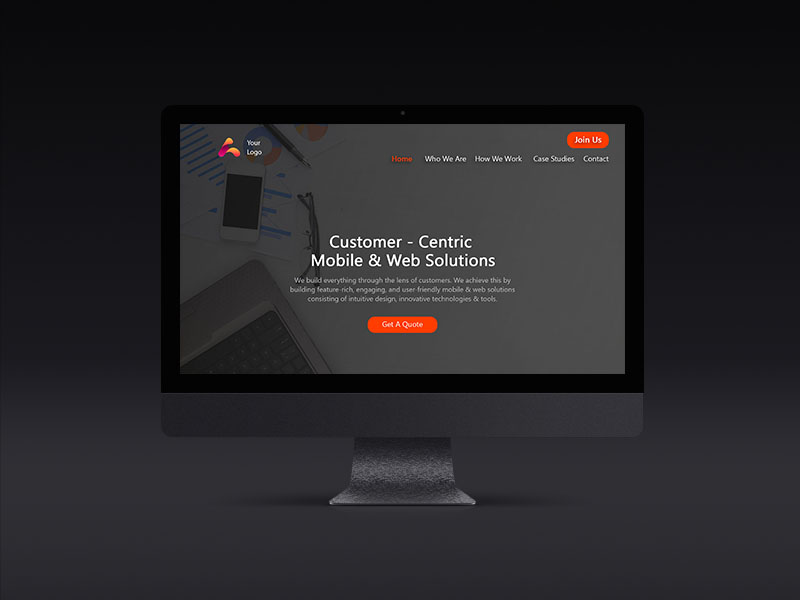The image portrays a slightly horizontally elongated black rectangle, featuring a computer-generated flat-screen monitor with a dubious drop shadow beneath it. The monitor displays text that reads: "Customer-centric mobile and web solutions. We build everything through the lens of customers. We achieve this by building feature-rich, engaging, and user-friendly mobile and web solutions. Continuing the intuitive design consisting of intuitive design, innovative technologies, and tech." The text appears with poor resolution.

Centrally located on the screen is a bright red button with white font that reads "Get a Quote". The background image resembles a photograph of a desk topped with a computer and a phone on the left side. The top left corner of the screen features the text "Your Logo" in white, while the top right corner has "Join Us" in a bright red-orange hue, similar to the "Get a Quote" button. Below this, a navigation menu with the options "Home," "Who We Are," "How We Work," "Case Studies," and "Contact" is displayed.